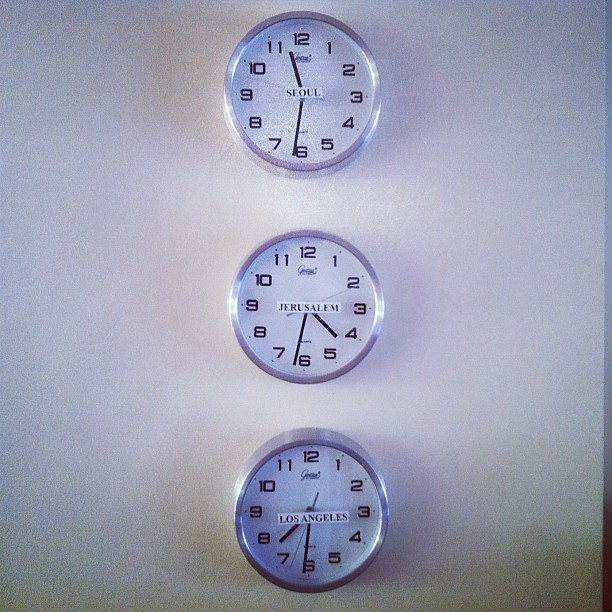The photograph depicts three identical silver-rimmed clocks with white faces and black hands and numbers, vertically aligned on a pristine white wall. Each clock bears an oblong sticker at its center, indicating different international cities. The top clock is labeled Seoul, marking the time at approximately 11:30. The middle clock is labeled Jerusalem, showing around 4:30. The bottom clock is labeled Los Angeles, with the hands positioned near 7:30. The clocks are evenly spaced and devoid of any second hands, except for thin black minute and hour hands. The simplicity of the background and the arrangement emphasizes the uniformity and purpose of the time display.